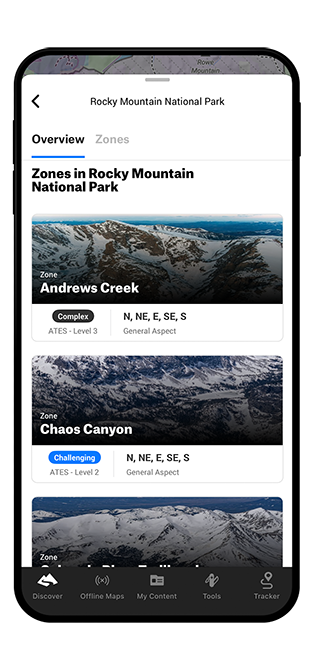This image is a screenshot from a mobile device displaying a page titled "Rocky Mountain National Park." At the top of the screen, centered and in bold black text, the title reads "Rocky Mountain National Park," with each word capitalized. To the left of the title, there is a black arrowhead icon pointing to the left. Below the title, two tabs are visible: the first tab, "Overview," is in bold black text with a blue underline indicating it is currently selected, while the second tab, "Zones," is in bold light gray text. A thin light gray divider line separates these tabs from the content below.

The first header, written in bold black text, reads "Zones in Rocky Mountain National Park." Below this header, there is a banner image depicting a snowy mountainous landscape, which may include a body of water or the blue sky in the background. In the bottom left corner of this image, small white text labels it as "zone." Below this, in larger bold white text, the caption reads "Andrews Creek."

Further down, the page features another section with a white background. On the left side, there is an oval shape with a dark gray background containing the word "Complex" in white text. Underneath this oval, small gray capital letters spell out "ATES - Level 3." A vertical gray line divider separates this section from the right side. On the right, in bold black text, several uppercase letters indicate directions: "N, NE, E, SE, S." Below this, small gray text reads "General aspect."

The content continues with another banner image of a snowy mountainous region, this one featuring more gray tones. In the bottom left corner of this image, small white text again labels it as "zone." Below this, in larger bold white text, the caption reads "Chaos Canyon."